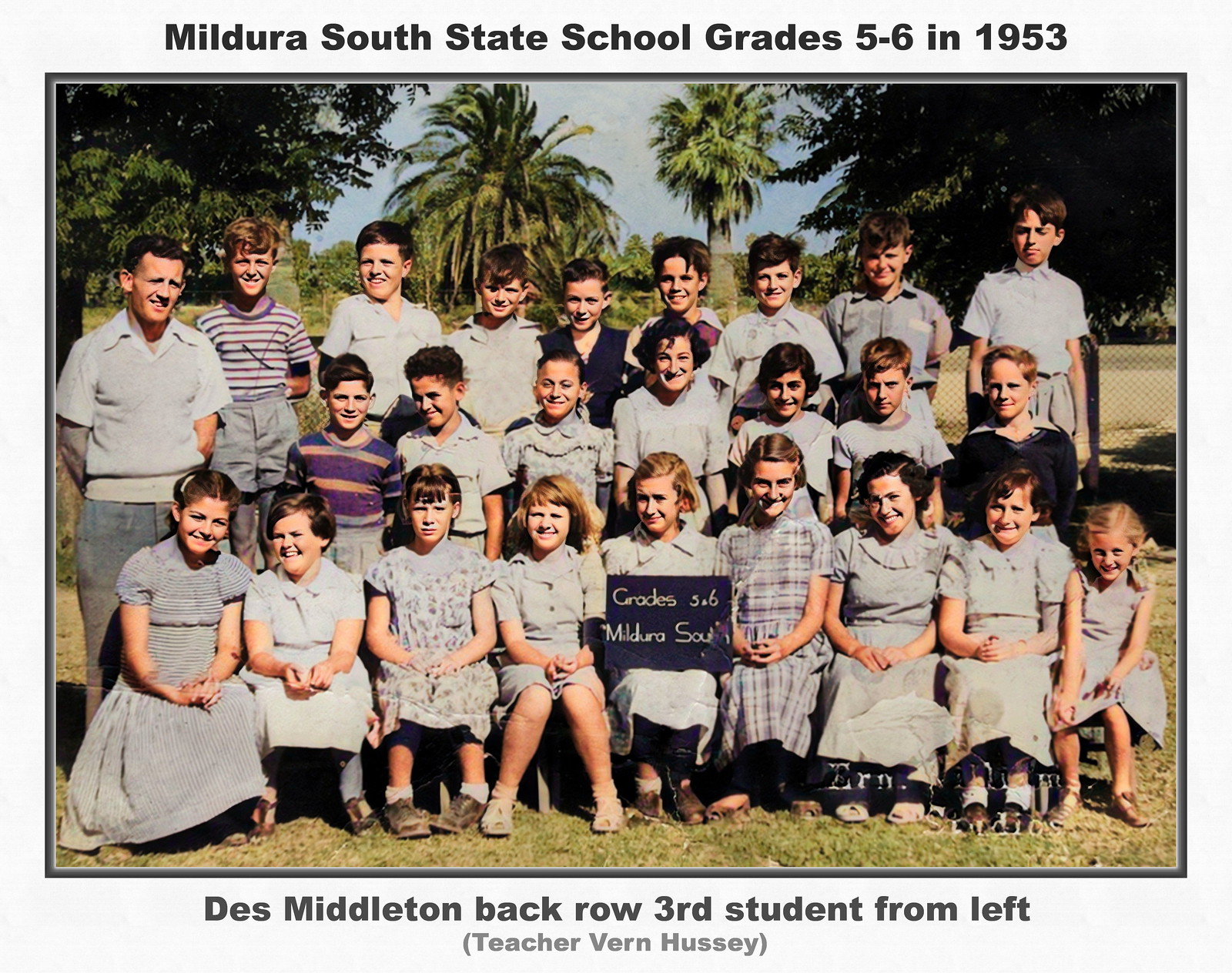This black-and-white photograph, possibly from 1953, depicts three rows of children from Mildura South State School, specifically grades 5-6. The image is framed with a light blue border, with "Mildura South State School Grades 5-6, 1953" written at the top. At the bottom, a caption indicates the presence of "Des Middleton, back row, third student from left" and identifies the teacher as "Vern Hussey."

The backdrop features palm trees and a clear blue sky, indicating an outdoor setting. The children are arranged in three rows: the front row is composed entirely of girls sitting and wearing dresses, while the middle row has a mix of girls and boys, with the children seated. The back row, which appears to consist entirely of boys and includes taller children, is standing. The teacher, a male named Vern Hussey, stands on the left side of the back row.

The students predominantly wear gray outfits, with a few exceptions of different colors. A notable feature of the photograph is a girl in the middle of the front row holding a chalkboard sign that reads "Grades 5-6 Mildura South." The image, though slightly faded, offers a nostalgic glimpse into a mid-20th century school setting.